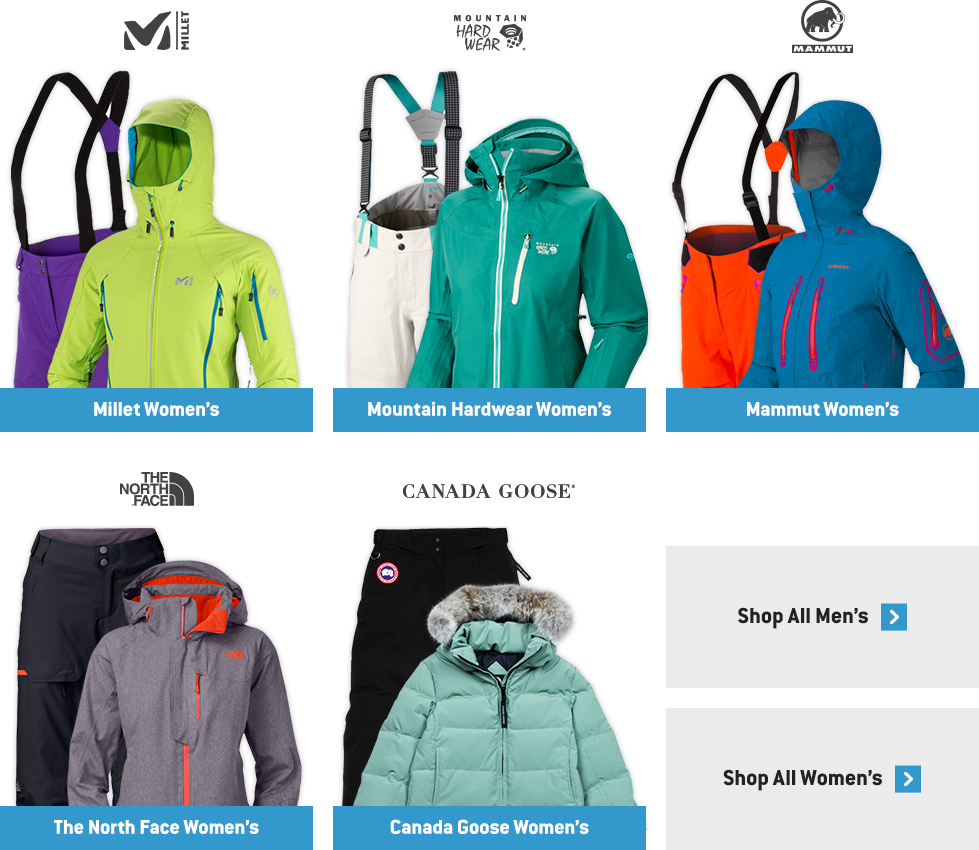The image showcases an outdoor retail clothing page featuring a selection of winter coats and snow pants. There are five complete sets displayed, with three sets on the top row and two sets below.

- **Upper Left Corner:** A green coat paired with purple snow pants from the brand Malay.
- **Center Top:** A light blue coat paired with white snow pants by Mountain Hardwear.
- **Upper Right Corner:** A dark blue coat with pink zippers matched with orange snow pants from Mammut, identifiable by their wooly mammoth symbol.
- **Lower Left Corner:** A purple coat with darker colored snow pants from The North Face.
- **Lower Right Corner:** A light blue coat with a furry collar accompanied by black snow pants from Canada Goose Women's.

Additionally, two selection boxes are stacked on top of each other to the right of the coat displays. The top box reads "Shop All Men's," and the bottom box reads "Shop All Women's."